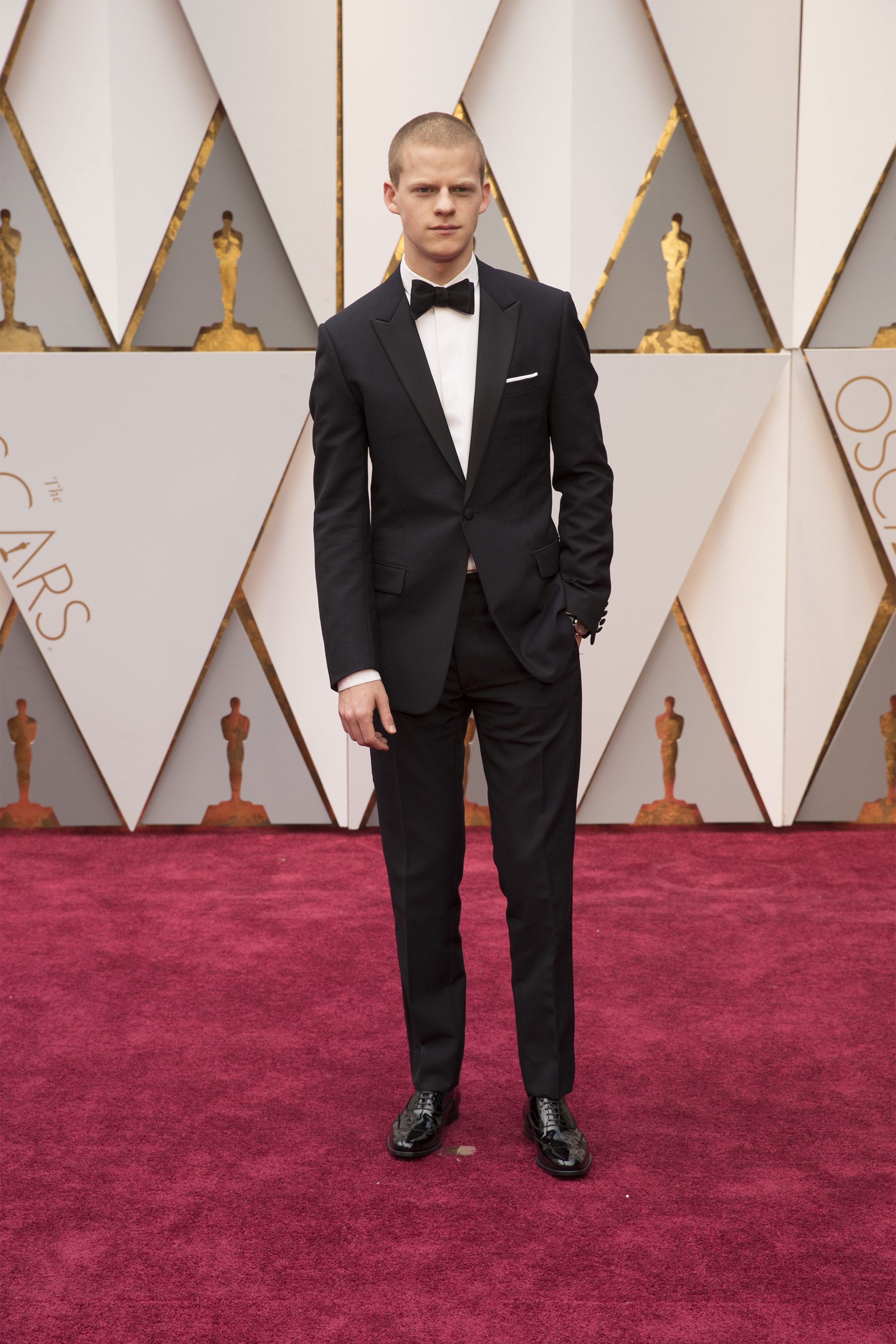A sharply dressed young man is striking a pose on the red carpet at the Oscars. He is wearing an elegant black suit, which might be a tuxedo, complete with a black jacket and matching trousers. His polished black shoes gleam under the lights. The outfit is complemented by a black bow tie and a white pocket square tucked into the breast pocket of his black dress shirt, under which he wears a crisp white undershirt. His hair is styled in a neat buzzcut, adding to his polished appearance. The backdrop features a wall adorned with the Oscars logo and golden designs, framing his poised stance perfectly for the photograph.